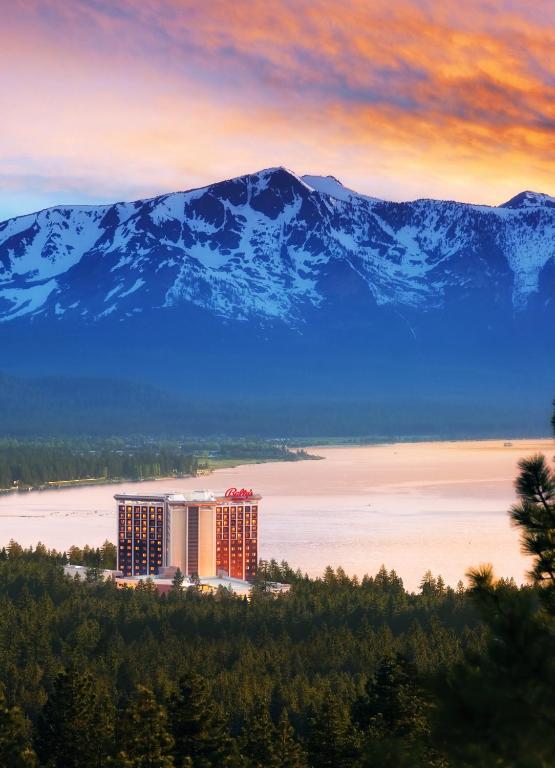This vibrant photograph, taken in a vertical and colorful format, captures a serene and expansive natural vista. Dominating the background is a majestic snow-capped mountain range partially veiled under an amber sky, with hints of blue peeking through the clouds. In the middle ground, nestled among thick layers of verdant forest, is the prominent Bally's Hotel, identifiable by its distinctive architecture and the red Bally's logo. The hotel structure showcases a captivating color gradient, transitioning from pink in the center to purple on the right side, and orange on the left. The building's white facade gleams with golden windows and red-topped valleys. The foreground reveals a dense canopy of treetops, leading down to a tranquil lakeshore that resembles a beach, lending a picturesque quality to the resort and its natural surroundings. This image beautifully combines elements of natural beauty with a touch of human sophistication, all bathed in the warm hues of an evening sky.